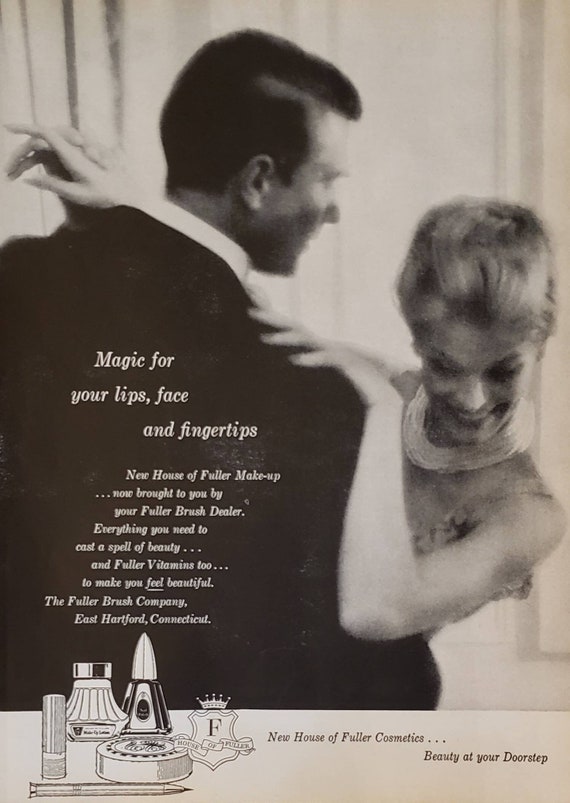The image is a vintage black and white ad featuring a man and a woman dancing. The man is dressed in a black suit with a white collared shirt and has brown hair, while the woman, with her blonde hair tied up, is wearing a strappy light-colored dress and a thick white necklace. She's smiling and looking down, with one arm around the man's neck and the other resting on his shoulder. The ad showcases a message on the back of the man's suit that reads, "Magic for your lips, face, and fingertips. New House of Fuller Makeup, now brought to you by your Fuller Brush dealer. Everything you need to cast a spell of beauty, and Fuller Vitamins II to make you feel beautiful. The Fuller Brush Company, East Hartford, Connecticut." The image features a white rectangular border at the bottom with outline sketches of makeup products, including a lipstick case, a perfume bottle, a pencil-like item, and a circular makeup compact. Next to these sketches, it states, "New House of Fuller Cosmetics, beauty at your doorstep." The overall aesthetic of the ad, characterized by its artistic, slightly out-of-focus charcoal drawing style, evokes a nostalgic vintage vibe, possibly from the 1960s.